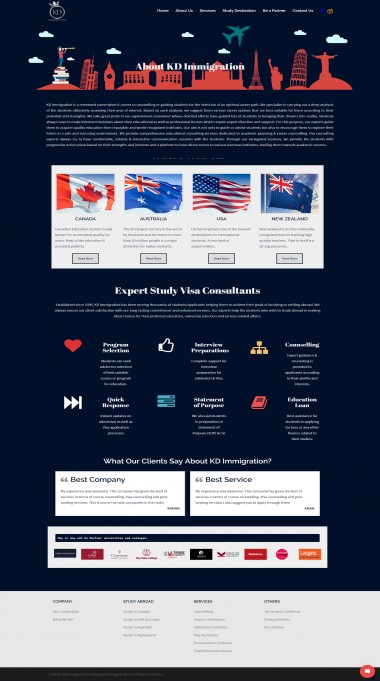The screenshot showcases a vibrant and informative promotional image for KD Immigration. At the center, bold text prominently reads "KD Immigration," surrounded by an illustration featuring iconic landmarks such as the Eiffel Tower and the Statue of Liberty. Beneath this central text, a detailed paragraph written in white text provides additional information. Following the paragraph, a row of national flags representing Canada, Australia, the United States, and New Zealand spans across the image, emphasizing global reach.

Further down, the phrase "Expert Study Visa Consultants" is displayed, complemented by an array of symbols including a heart, a fast-forward button, a thumbs up, various bar graphs, and a book, symbolizing the comprehensive support offered. At the very bottom, the section titled "What Our Clients Say About KD Immigration" presents two client reviews, attesting to the service’s credibility. Lastly, a small chat option button is visible in the bottom right corner, inviting users to engage directly for more information.